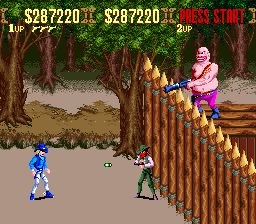This detailed image captures a scene from a retro-style, pixelated video game reminiscent of 1990s arcade graphics. At the top of the screen, the score is displayed in yellow as "$287,220," repeated twice, while on the far right, "PRESS START" is highlighted in red capital letters. The background features a forest with green, deciduous trees, followed by a sandy beige area transitioning into a darker brown section bordered by rocks. The scene is set at an old-time wooden fort with pointed posts and picket fences. 

Within the fort stands a bare-chested, overweight villain with a European appearance, wielding a blue gun and dressed in purple wrestling tights and boots. Shooting over the fence, this character threatens the two cowboys positioned outside the blockade. One cowboy, clad in green jeans, a white shirt, and a green hat, has just fired a green projectile from his pistol towards the other cowboy, who sports a blue shirt, blue jeans, white pants, and a blue hat. An orb—possibly indicating the projectile's path—hangs between them. The visual setting enriches the historical Western duel feel while retaining the charm of early video game design.